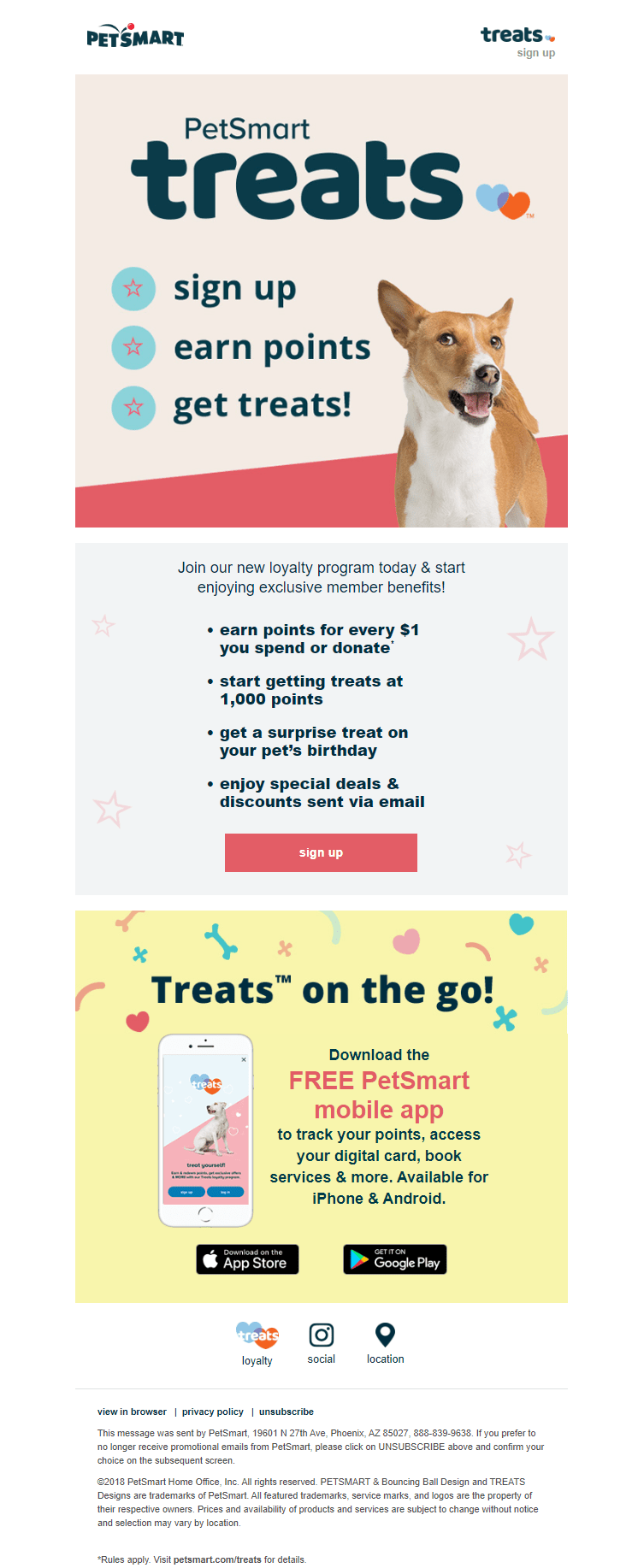This screenshot from the PetSmart app showcases an advertisement for PetSmart Treats. At the top left, the PetSmart logo is prominently displayed, with the Treats logo and a "Sign Up" button to its right, all set against a clean, white background.

The main section of the ad is divided into three distinct boxes:

1. **First Box:** This section features the PetSmart Treats logo alongside a call to action to sign up for great treats. It showcases an image of a smiling, fawn-colored dog with a white chest. The background is predominantly cream-colored with a red section at the bottom angled upwards.

2. **Second Box:** Continuing with the cream-colored background, this section invites users to join the new loyalty program with the line, "Join our new loyalty program today and start enjoying exclusive member benefits!" The benefits are listed in black font with four bullet points:
   - Earn points for every one dollar you spend or donate.
   - Start getting treats at 1,000 points.
   - Get a surprise treat on your pet's birthday.
   - Enjoy special deals and discounts sent via email.
   At the bottom of this box is a red "Sign Up" button.

3. **Third Box:** The final section has a yellow background and features the title "Treats on the Go." Small icons of dog treats and hearts are scattered throughout. This section promotes the PetSmart mobile app, noting that the app allows users to track points, access a digital card, book services, and more. The app is available for both iPhone and Android.

Overall, the ad effectively conveys the benefits of joining PetSmart's loyalty program and highlights the convenience of their mobile app.